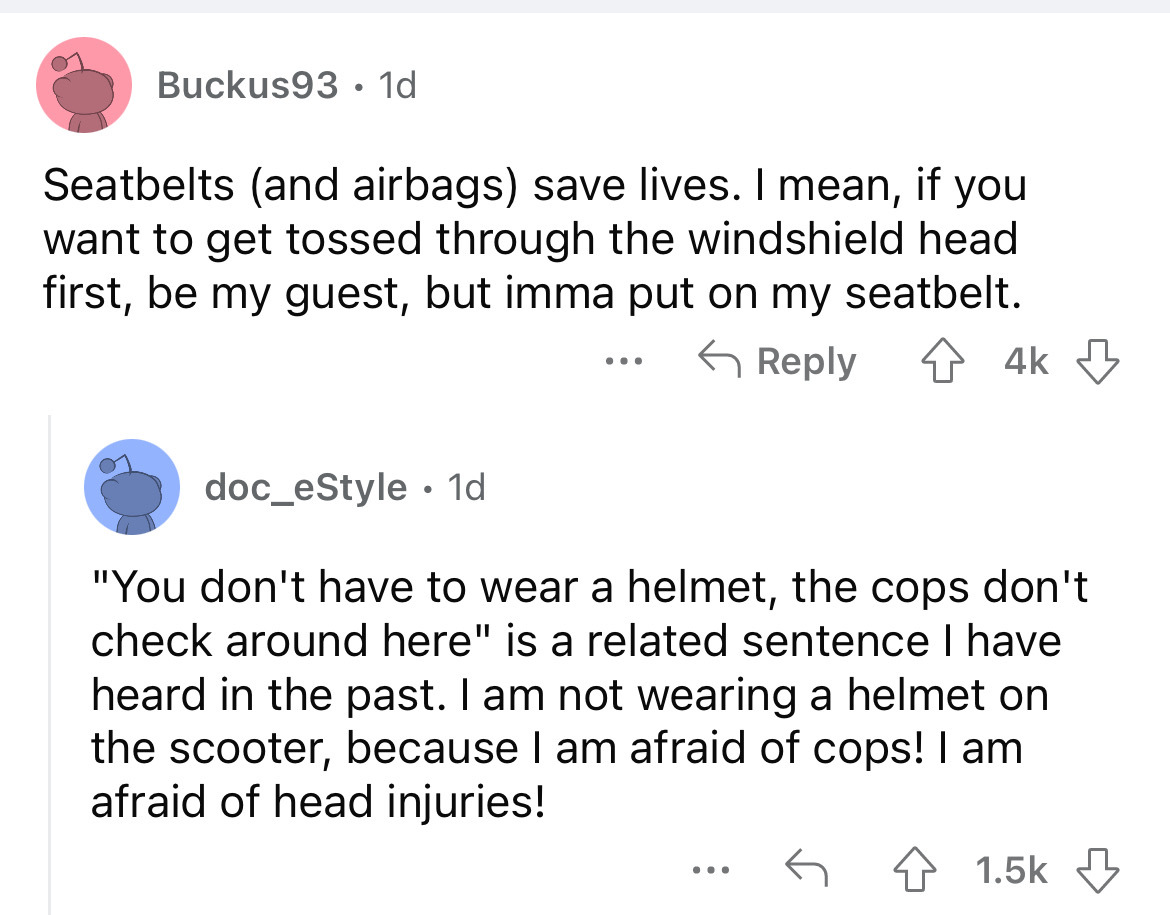The screenshot captures a text conversation between two individuals, identified by their unique avatars and usernames. 

At the top of the screen, an avatar displaying a small pink alien represents the user "Buckus 93." Next to the avatar is the label "1d," indicating the message was sent one day ago. Buckus 93 shares a firm stance on safety, saying, "Seatbelts and airbags save lives. If you want to get tossed through the windshield headfirst, be my guest, but I'm going to put on my seatbelt." This message has received options to reply or vote, with an upward arrow indicating it has garnered 4,000 upvotes.

Beneath Buckus 93's message is a slightly indented response from another user, "doc_e_style," whose avatar features a small blue robot. Their message is also labeled "1d," suggesting it was posted around the same time. Doc_e_style quotes a familiar, albeit reckless sentiment, and counters it with their own reasoning: "'You don't have to wear a helmet; the cops don't check around here,' is a related sentence I have heard in the past. I'm not wearing a helmet on the scooter because I am afraid of cops; I am afraid of head injuries." This message also has the options to reply or be voted on and has accumulated 1,500 upvotes.

The top of the screenshot displays a light gray row, but no additional information is provided beyond the interface elements for interaction and the content of these two messages.